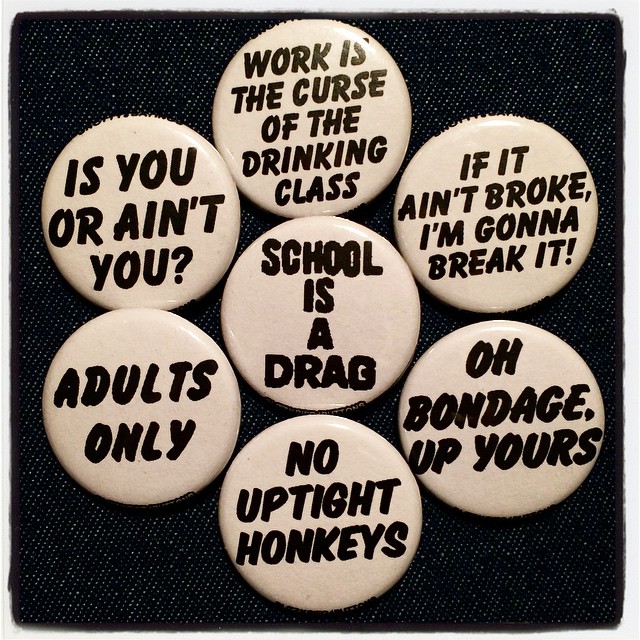The image displays a collection of seven white buttons with handwritten-style black text arranged on a black piece of denim. The buttons are positioned in a flower shape, with six forming a circle around a central button. Each button carries a different text: 

1. "Work is the curse of the drinking class"
2. "If it ain't broke, I'm gonna break it"
3. "Oh bondage up yours"
4. "No uptight honkies"
5. "Adults only"
6. "Is you or ain't you?"
7. (center) "School is a drag"

The overall composition combines the stark contrast of the white buttons and black text against the dark denim background, creating a visually striking and rebellious aesthetic.